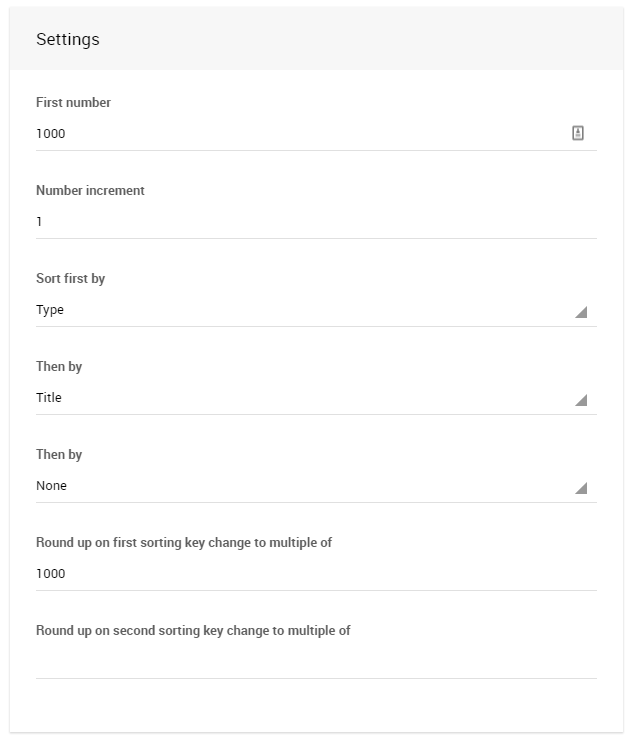This image depicts a screenshot of a settings box with various configuration options outlined in a structured format. 

At the very top, there's a light gray bar with the word "Settings" prominently displayed in black lettering. Below this bar, the settings are organized into distinct categories, each separated by thin gray lines.

1. The first setting is labeled "First Number" and shows the value "1,000" entered. To the right of this value, there is a small symbol.
2. Following this, the setting "Number Increment" has a value of "1" entered.
3. The next category, "Sort First By," has the option set to "Type." A small triangle icon pointing downwards on the right indicates this is a drop-down menu.
4. The subsequent setting, "Then By," is configured to "Title," with another drop-down triangle icon present on the right.
5. Another "Then By" category follows, with the option set to "None," alongside another drop-down triangle.
6. Moving forward, the setting "Round up on First Sorting Key Change to Multiple Of" has the value "1,000" entered.
7. Below this, the setting "Round up on Second Sorting Key Change to Multiple Of" appears, but no value is entered.

The settings box concludes at this point, maintaining a consistent structure with gray lines delineating each section.